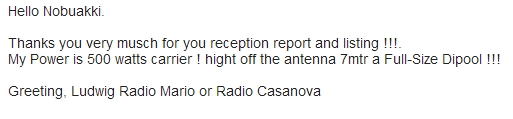The image is a white background with small, dark gray or black text, resembling a graphic or postcard typically used for reception confirmations. The text, marred with typos and grammatical errors, appears to be a message, possibly sent via ham or shortwave radio, and reads:

"Hello Nobuaki. Thank you very much for your reception report and listing!!! My power is 500 watts carrier. Height of the antenna is 7 meters, a full-size dipole. Greetings from Ludwig Radio Mario or Radio Casanova."